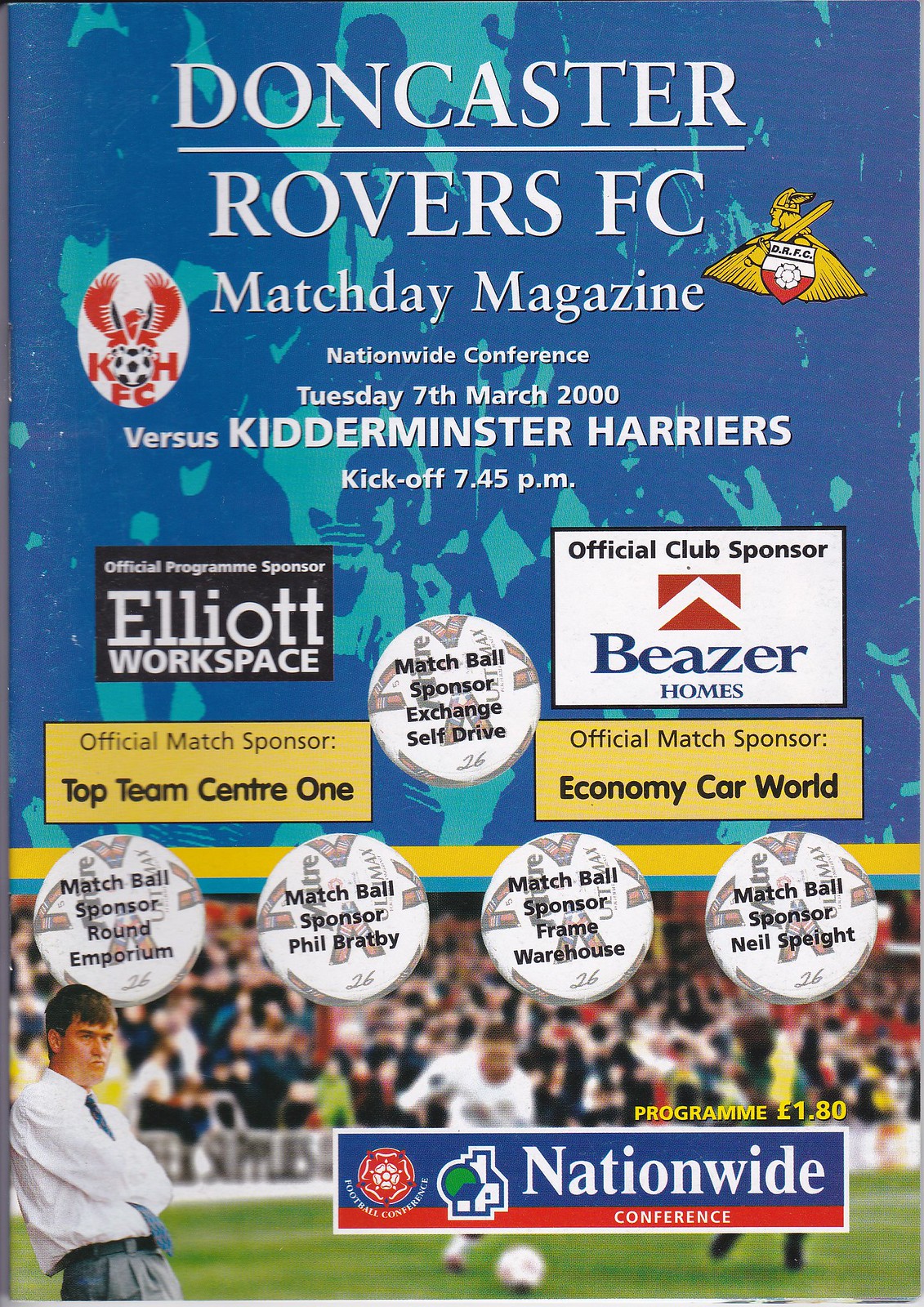This is the vividly colorful cover of the Doncaster Rovers F.C. Match Day Magazine for the Nationwide Conference held on Tuesday, March 7, 2000, against the Kitterminster Harriers, with a kickoff at 7:45 p.m. The background features an abstract blue and aqua pattern, which sets a striking stage for the array of information presented. Prominent at the top are the words "Doncaster Rovers F.C." and "Match Day Magazine" accompanied by a gold logo featuring a winged warrior with a sword and a white oval with "K.H.F.C." and a red wings creature.

The cover is populated with several inset commercials and advertisements: Official Program Sponsor Elliott Workspace, Official Club Sponsor Beezer Homes, Official Match Sponsor Economy Car World, and Official Match Sponsor Top Team Center One. Additionally, there are soccer balls featuring additional sponsors, including the Match Ball Sponsor Exchange Self Drive.

Occupying the bottom third of the cover is an out-of-focus image of the pitch with what appears to be fans in the stadium. To the left, a man dressed in a white shirt, gray trousers, and a green tie stands with arms folded, leaning slightly against a wall and looking right. The bottom right corner of the cover prominently displays "Nationwide Conference" in red and blue. The magazine price is listed as £1.80.